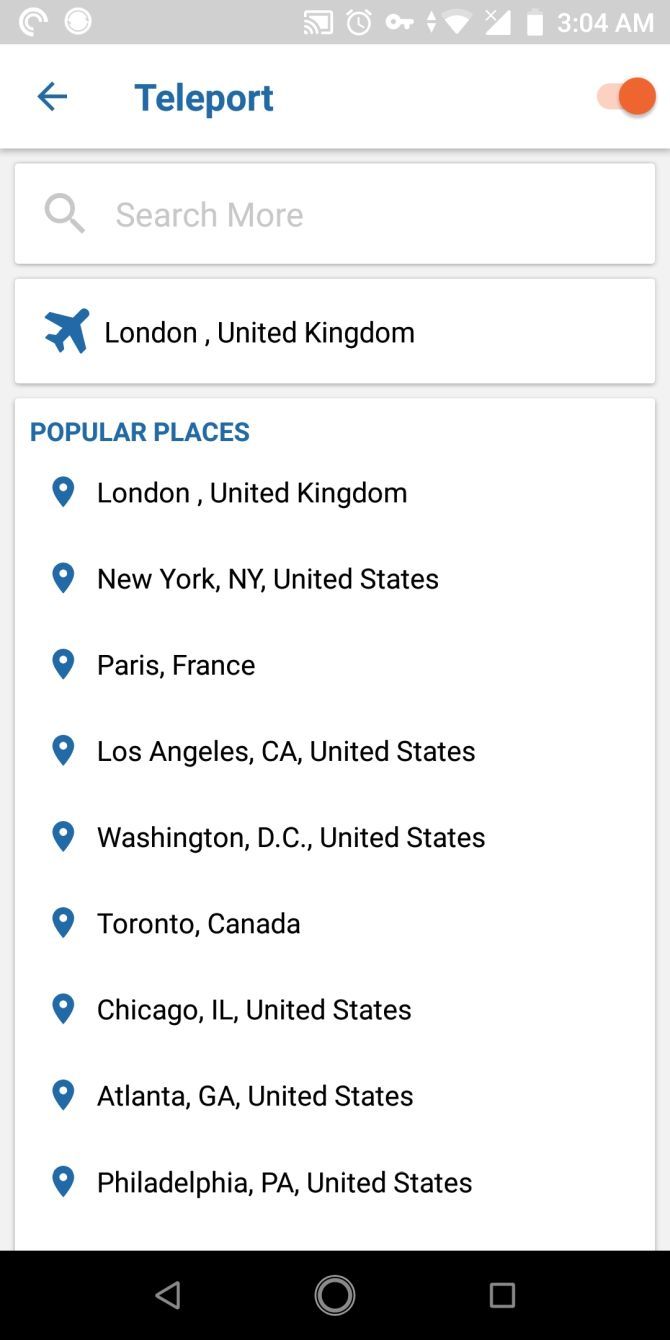The image features a screenshot of a smartphone displaying a travel or location-based app. At the top, there's a thin gray banner housing various status indicators. On the left, a white key icon and a home icon appear next to a digital clock. Near the center-right, there is an X symbol, typically indicating no cellular reception, followed by a mostly charged battery icon. 

Below this status bar is a navigation section. On the left side, a blue arrow points to the left, labeled "teleport." Adjacent to this is an orange circle.

The screen background is predominantly white, featuring three rectangular sections arranged vertically. The first section contains a gray magnifying glass icon with the text "Search and War." The second section depicts a blue airplane ascending, accompanied by the text "London, United Kingdom." The final section highlights popular destinations, displayed in bluish-gray box tails, listed in black text as follows: 

1. London, United Kingdom
2. New York, New York, United States
3. Paris, France
4. Los Angeles, California, United States
5. Washington, D.C., United States
6. Toronto, Canada
7. Chicago, Illinois, United States
8. Atlanta, Georgia, United States
9. Philadelphia, Pennsylvania, United States